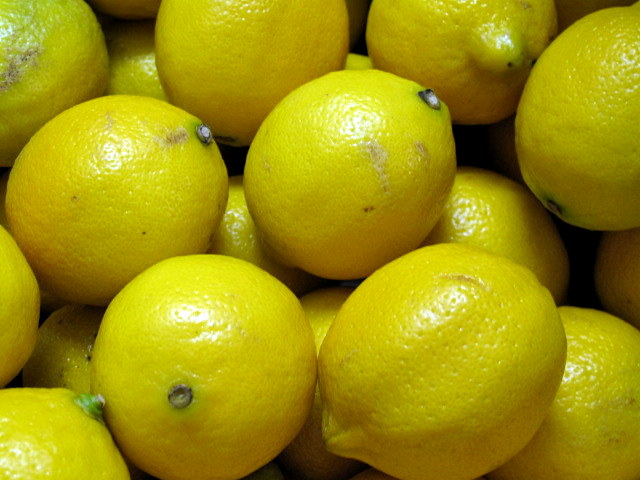This high-quality close-up photograph captures a pile of around 15 lemons, taken from a bird's eye view. The picture showcases an array of whole, shiny lemons, their waxy yellow skins glistening under the light shining from above. The front of the image prominently features two whole lemons, with the one on the left displaying a visible stem attachment point. Among the lemons, there are occasional green and brown blemishes, indicating some bruising. Notably, towards the upper right corner, there is a lemon with a distinctive nipple-like protrusion. The lemons are stacked in layers, with some partially hidden, creating a dense, vibrant composition.